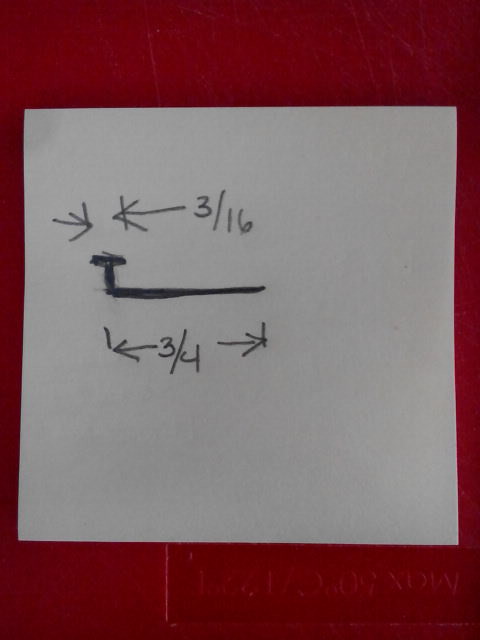This image features two hand-drawn arrows on a sticky note, each pointing at different measurements. The first arrow points to a notation of "3/16," indicating a length of 3/16 of an inch. The second arrow directs attention to a measurement labeled "3/4," signifying 3/4 of an inch. The sticky note serves as a makeshift diagram or reference, illustrating these fractional inch measurements with precision and clarity.